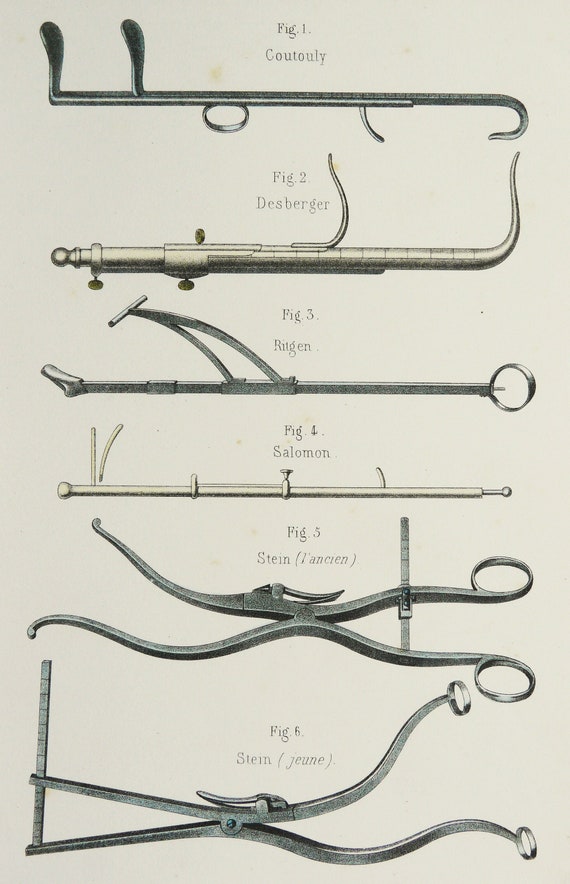This image is an illustration of six detailed, silver, metal tools likely of medical, possibly dental or surgical nature, shown on an off-white background. Each of the six tools is labeled with a figure number and name:

1. **Figure 1, Cotonly**: This tool features two paddle-like levers on the left and a circle in the bottom middle, presumably for a finger, with a hooked end on the right. 
2. **Figure 2, Desperger**: Comprising a plunger on the left side, two hooks—one in the middle, one at the far right—and several turning knobs, this tool appears to be adjustable.
3. **Figure 3, Rugen**: This instrument has a loop on the bottom right, a protruding paddle-like lever on the left, and a central sliding piece that forms a V-shape.
4. **Figure 4, Salomon**: A straightforward, linear tool with small spherical ends and subtle screws for potential adjustment.
5. **Figure 5, Stein**: Resembling scissors, but with curved, wavy blades that culminate in small balls rather than sharp edges.
6. **Figure 6, Stein**: Another scissors-like tool with circular finger holes and a ruler-like protrusion on the left.

All tools exhibit intricate, multi-functional designs with various hooks, loops, paddles, and adjustment mechanisms indicating their specialized uses.